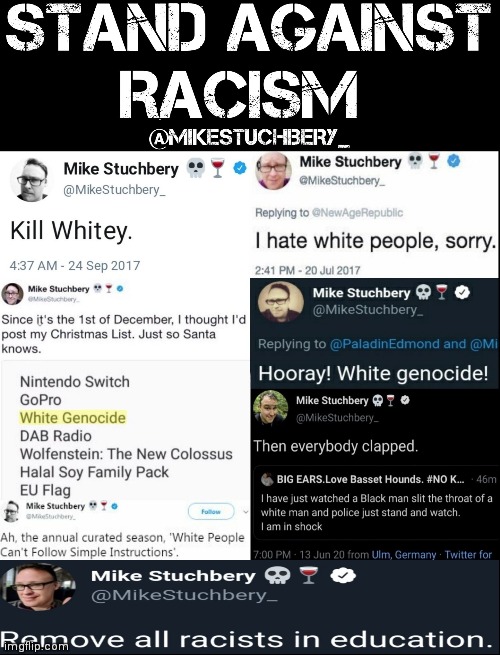The image is a collage of various screenshots from what appears to be Twitter, now known as X. At the top of the collage, there is a prominent message on a black background with white text that reads "Stand Against Racism," credited to the user Mike Stuckberry, indicated by the handle "@MikeStuckberry_". The collage features multiple tweets from the same user, Mike Stuckberry, some of which contain inappropriate comments. The backgrounds of the tweets toggle between black and white, and the profile picture of the user varies in some of the screenshots. One notable tweet, dated for the first day of December, states, "I thought I’d post my Christmas list just so Santa knows." The collage is noted to have originated from the website imgflip.com.